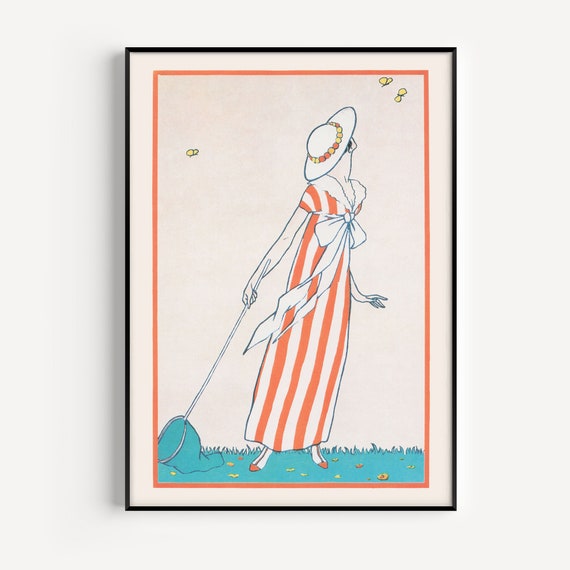This piece of art, framed in a thin black frame with a white mat and an inner coral outline, hangs on a pristine white wall. The artwork depicts a woman standing on green grass, wearing a coral and white striped dress adorned with a flowing white bow in the center. She is delicately shod in small coral shoes, and her attire is completed by a white hat embellished with orange and yellow beaded pieces around its inner edge. In her right hand, she holds a butterfly net, which blends into the grass below her. The woman gazes upward, towards three yellow butterflies fluttering in the sky—two on the top right and one on the left. The scene captures her poised in a moment of serene anticipation, perhaps ready to catch the vibrant butterflies. The detailed line-style drawing adds a delicate touch to the overall composition.